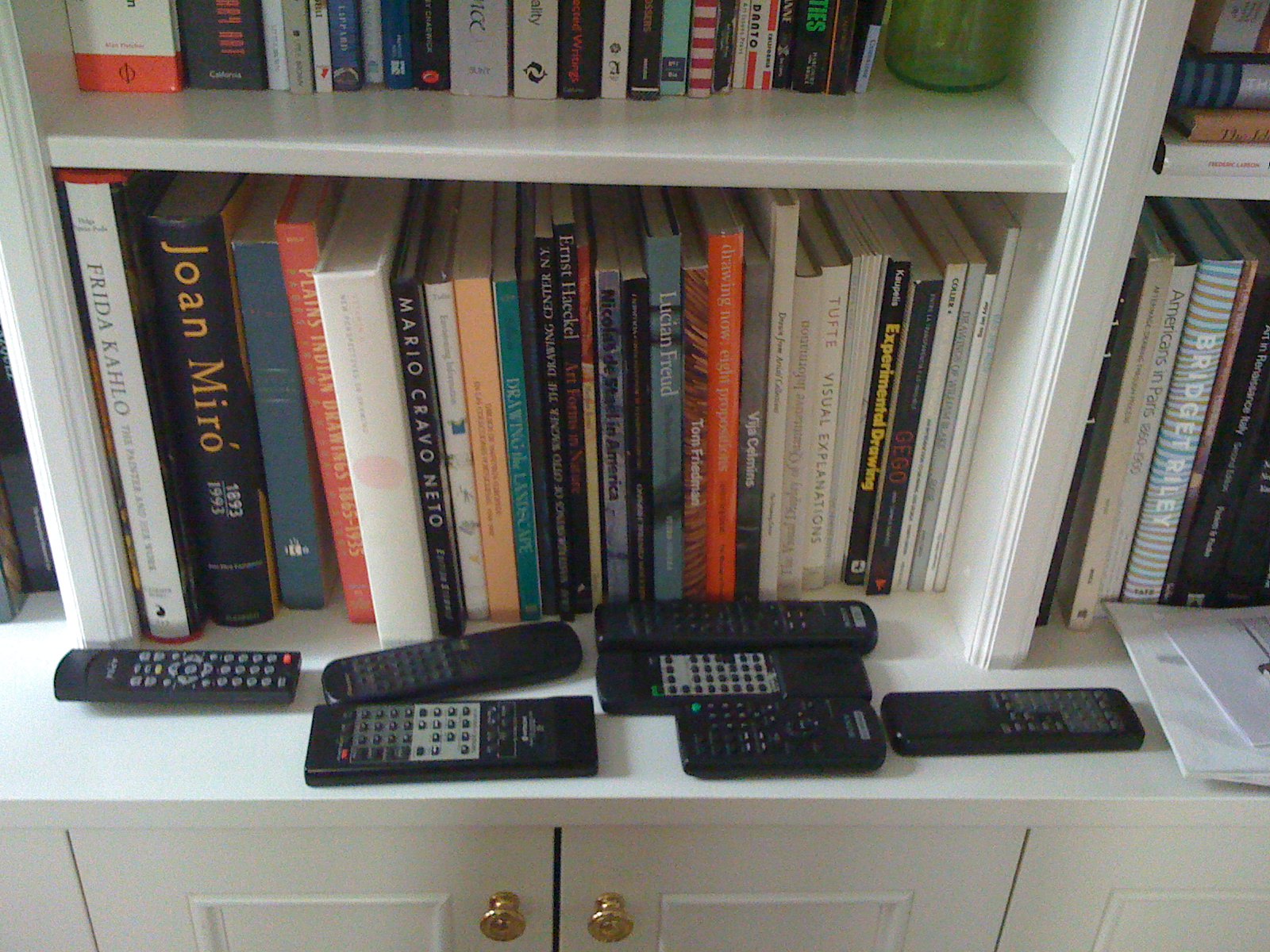The photograph features a white bookcase with four shelves filled with books, some of which include titles such as "Frida Kahlo," "Joan Miró," and "Mario Cravo Neto." The top shelf is fully visible with a row of books, while the other shelves have partially visible books due to foreground objects. The base of the bookcase extends slightly outward and features cabinet doors with gold handles, which are open to reveal additional storage space. 

On the middle shelf, seven black remote controls, each with various red and green buttons, are lined up neatly. These remotes are of different models and designs, evoking a sense of old-fashioned VCR or 1980s technology. Among them, two remotes appear identical, sporting black and gray colors. There is also a distinguishable long remote with a prominent red button. Scattered papers lie to the right side of the remotes, and the overall scene includes hardcover and softcover books of various colors—orange, green, black, yellow, and white. The detailed arrangement of remotes and books forms a unique visual juxtaposition against the clean white backdrop of the furniture.